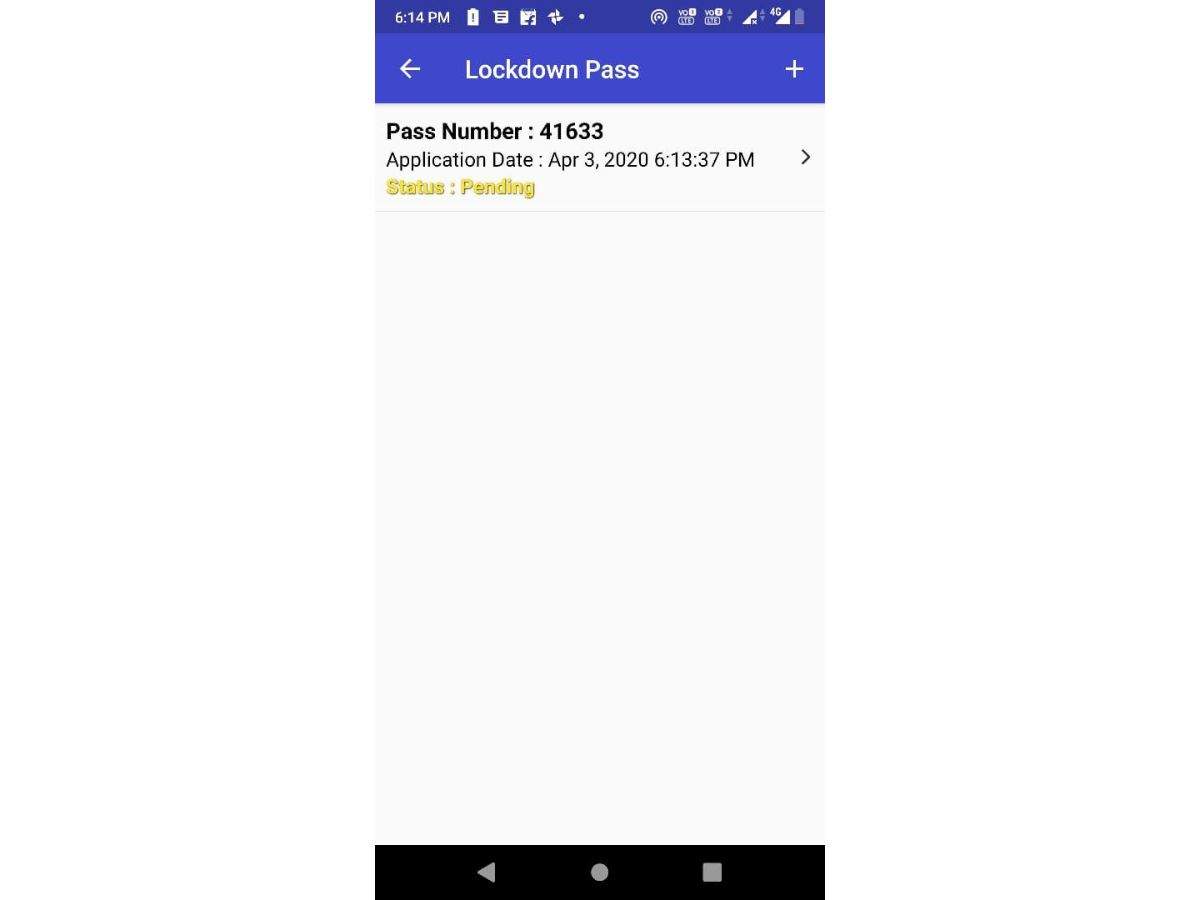This image is a screenshot from a cell phone displaying various status icons and an important notification. At the top left corner, the time is displayed in white against a dark blue background, indicating it is 6:14 p.m. To the right, there's a white battery icon with an exclamation point, signaling a low battery. Next to the battery icon, there are several application icons and indicators, including a text box, a Facebook icon, and another icon featuring four small symbols followed by a dot.

Further along, there is a Wi-Fi symbol, and next to it, indicators that appear to show network data status labeled as "LTE" for both "VO3" and "VO2," along with a triangle and an 'X' symbolizing a network issue on a 4G network. Additionally, there is another triangle icon, and arrows pointing up and down indicating data usage, further confirming network activity.

Below this status bar, in a lighter blue banner with a left-pointing arrow, the text "Lockdown Pass" is prominently displayed in white, with a white plus sign to the right of it. Beneath the banner, in bold black text, is the pass number: "41633." The application date, in standard black text, reads "April 3rd, 2020, 6:13:37 p.m." Following this, there is a yellow status indicator in bold text that states, "Status: Pending."

This screenshot likely pertains to a digital lockdown pass application, detailing its status and application timestamp amid various phone status indicators.